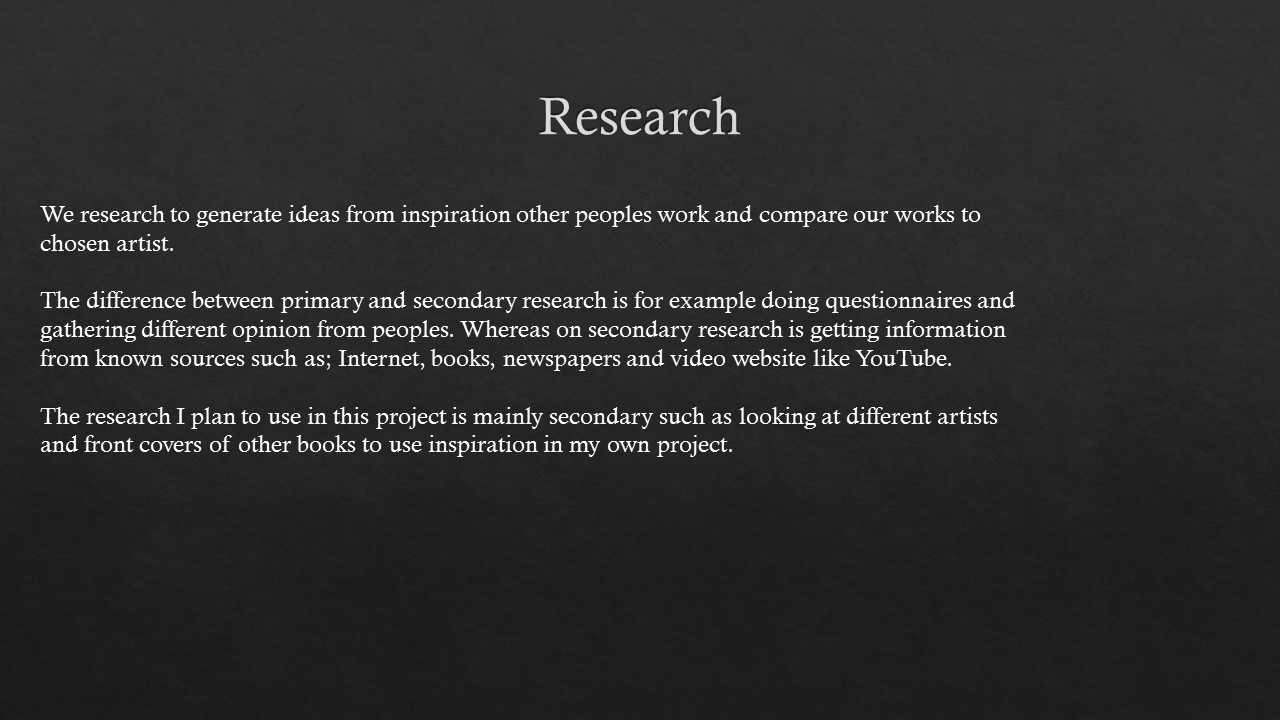The image features a black background with white text, displaying three paragraphs centered around the topic of research. At the very top, in large font, is the word "Research." Beneath it, in smaller text, it states: "We research to generate ideas from inspiration, other people's work, and compare our works to chosen artists. The difference between primary and secondary research is, for example, doing questionnaires and gathering different opinions from people. Whereas secondary research involves getting information from known sources such as the Internet, books, newspapers, and video websites like YouTube. The research I plan to use in this project is mainly secondary, such as looking at different artists and front covers of other books to draw inspiration for my own project." The text appears to aim for a professional tone but is casually captured, suggesting that the author's first language may not be English. There are no other objects or pictures within the image.